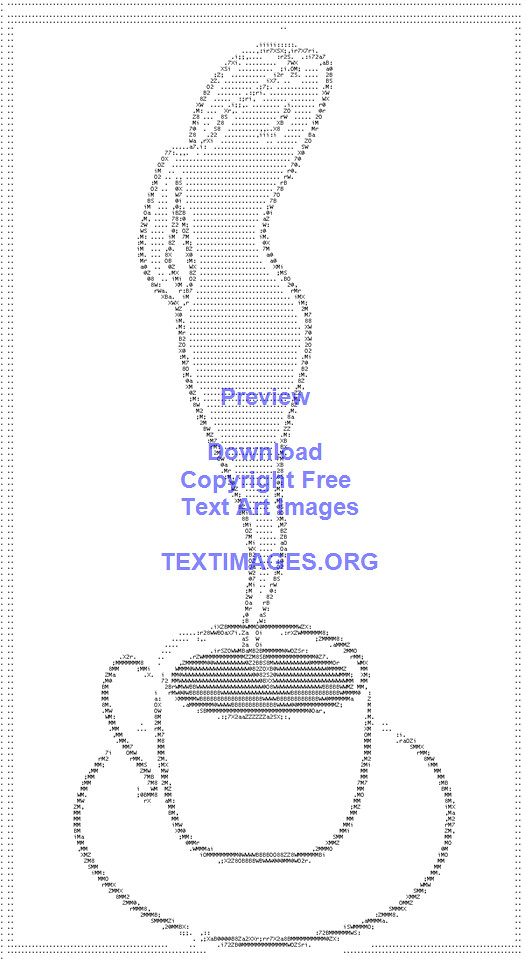A digital artwork from textimages.org features a stylized coffee cup filled with a dark liquid, likely coffee, sitting on a saucer. Rising from the center of the cup, steam forms the graceful figure of a young woman with long hair. She strikes a seductive pose with one arm down by her side and the other arm wrapped over her head, her face resting near her armpit. The entire image is created using text or characters, and is overlaid with blue text that reads, "Preview. Download copyright-free text art images at textimages.org."